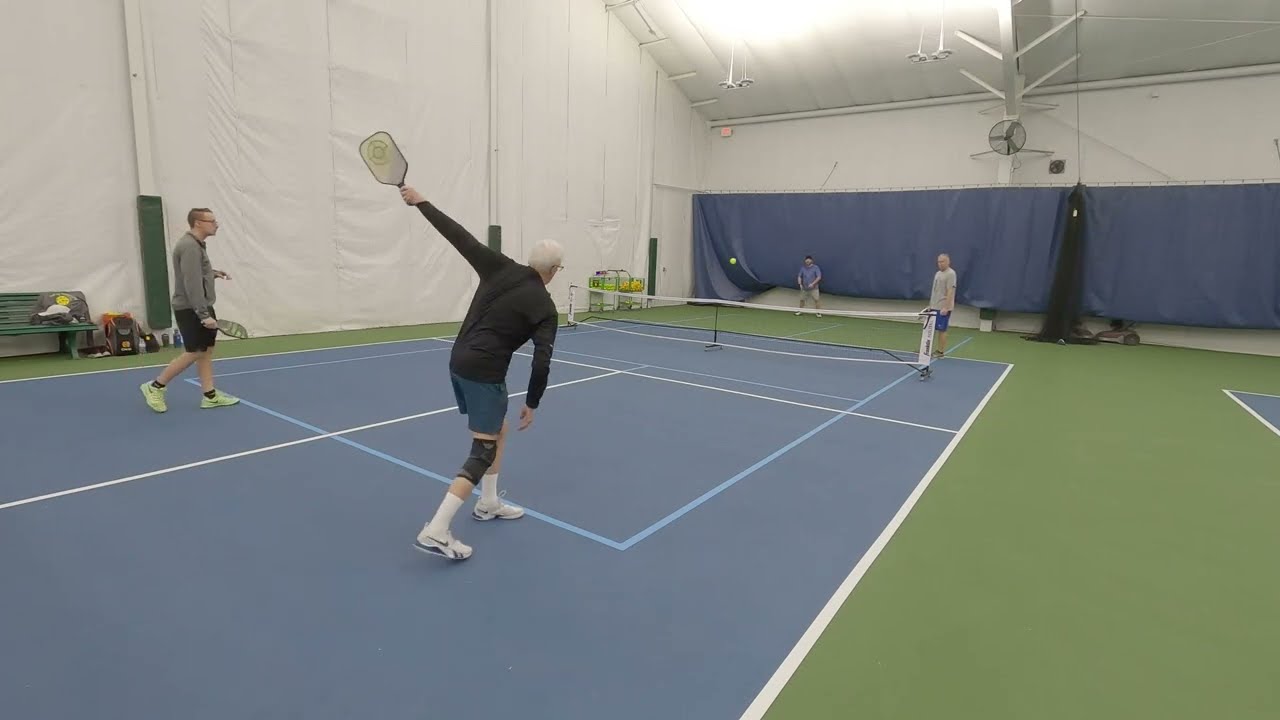This full-color, horizontally rectangular photograph captures an indoor scene in an athletic facility with white walls and patches of blue tarp. The lighting is ample, with some natural light filtering from the ceiling and additional lights directly above the play area, illuminating a well-defined blue court with white stripes bordered by a green floor. The scene depicts a doubles pickleball match. In the foreground, an older gentleman with gray hair is prominently featured, wearing white shoes, socks, blue pants, a long-sleeve black top, and a knee brace on his right knee. He is partnered with a younger man dressed in a gray top and black shorts. On the opposite side of the net, also dressed for a pickleball match, are another two players: one in a blue shirt with gray shorts and the other in a gray shirt with blue shorts. The net is a short, white-and-black design, and a yellow pickleball is caught mid-flight over the net, indicating an active serve, as the man on the right in the foreground has his paddle arm raised. White curtains hang along the side, and there's a noticeable container holding more yellow pickleballs in the back. The overall atmosphere suggests an engaging, well-lit indoor sports activity.